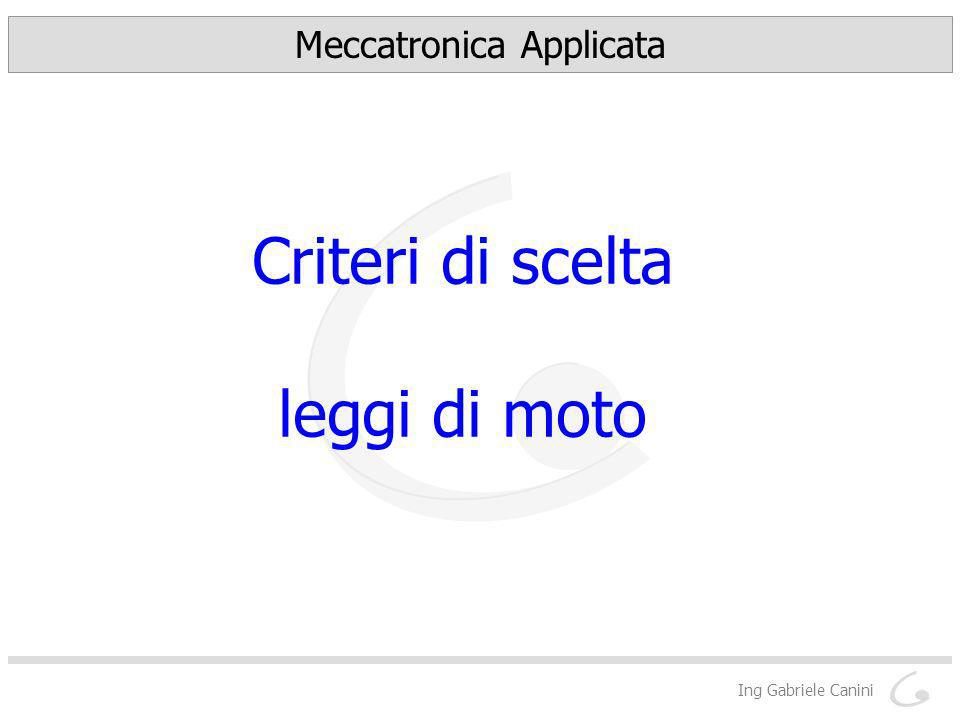The image features a minimalistic design with a clean white background. At the top is a narrow horizontal gray rectangle containing the title "Mechatronica Applicata" in black letters. Below this, centered in the main part of the image, are two lines of text in blue letters; the first line reads "Criteri De Scelta," and the second line reads "Leggi Di Moto." Behind this text, there is a gray watermark logo shaped like a 'C' with a circle at the top end of the 'C.' At the bottom of the image, a thin black horizontal line stretches across the width of the image, beneath which is the name "Ing. Gabriele Canini" next to the same gray 'C' shaped logo.